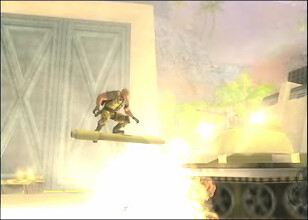The image depicts a scene from an older video game, potentially from the PlayStation 2 era, featuring a soldier in camouflage clothing standing on the barrel of a green tank. The soldier adopts a stance similar to that of someone riding a surfboard, slightly crouched. Bright spotlights illuminate the scene, which is set against a backdrop featuring palm trees and a vivid, pink sunset sky. To the left of the frame, two green doors with large "X" patterns are visible on a white wall, partially shrouded in flames. The setting appears tropical, evidenced by the palm trees, and the background also includes a starry sky. The bright light in the center gives the impression of an explosion or intense illumination, further indicating action or combat within this video game scenario.